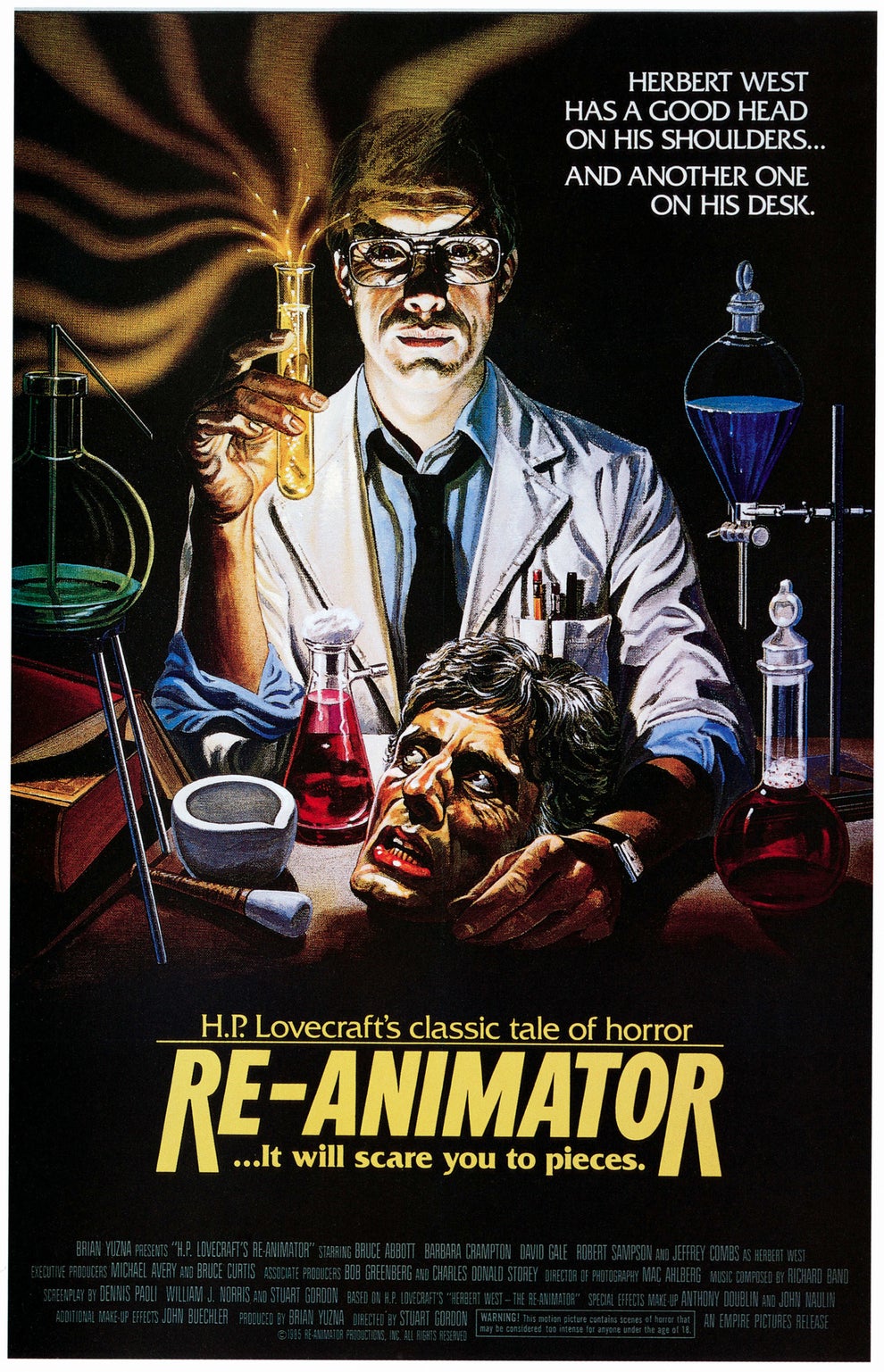This movie poster for "Re-Animator," based on H.P. Lovecraft's classic tale of horror, features a detailed color illustration with a dark, ominous background. The central figure is a scientist, illuminated eerily from below, accentuating his intense expression as he sits at a cluttered lab bench. He wears large square glasses, a white lab coat with pockets stuffed full of pens and pencils, and a blue Oxford button-down shirt with rolled-up sleeves and a loose, dark tie. In his right hand, he holds a beaker streaming amber-colored fumes, while his left hand, adorned with a wristwatch, rests next to a severed head on the desk — a head that vaguely resembles Al Pacino and appears to be alive, looking back at him. Surrounding the scientist are several pieces of laboratory equipment, including Erlenmeyer flasks filled with reddish liquids, other boiling-type flasks on stands, a mortar and pestle, and various clamps and lab apparatus. 

The top of the poster reads in white lettering, "Herbert West has a good head on his shoulders... and another one on his desk." At the bottom, in large bold yellow font, it announces "H.P. Lovecraft's classic tale of horror, Re-Animator" with the tagline "It will scare you to pieces." Along the bottom of the poster are the typical movie credits in smaller white lettering, which are not legible.